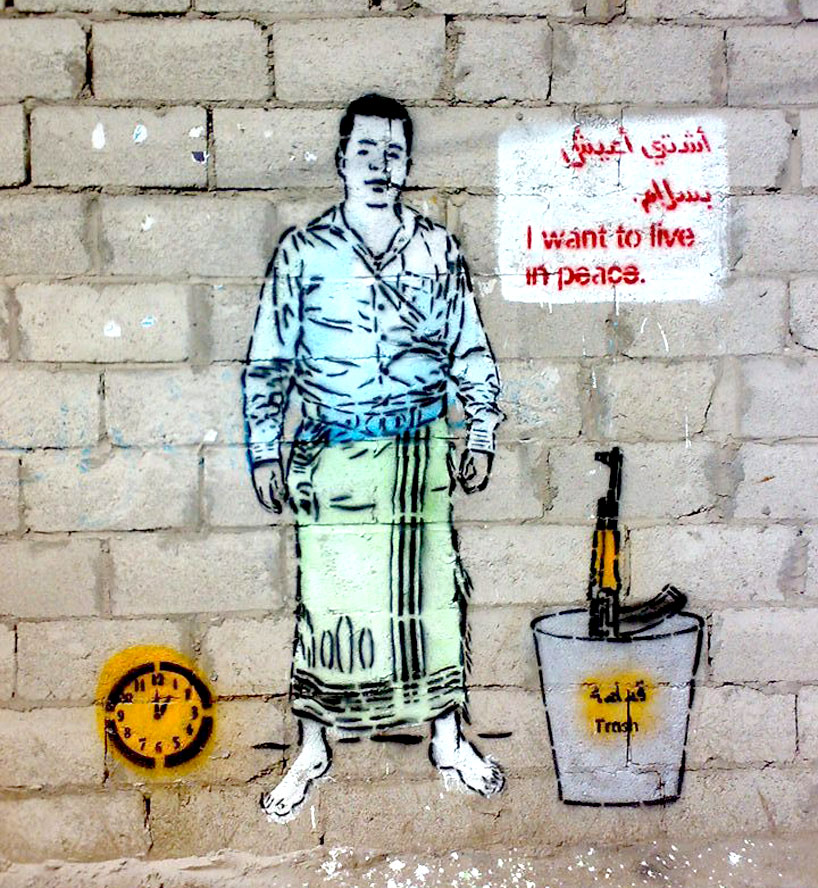The image depicts a striking piece of street art graffiti set against a gray cinder block wall, which appears to be inspired by the style of Banksy. Central to the artwork is an animated depiction of a man with pale skin, black hair, and barefoot. He is wearing a light blue shirt or jacket and a green towel with black designs around his waist. The man is positioned in the middle of the wall.

To his right, on the lower left of the image, there is a clock with an orange background, black numbers, and hands, showing the time as one o'clock. On the man's left side, towards his legs, a trash can is depicted, labeled "trash" and containing a rifle, possibly a Kalashnikov. 

In the top right corner of the wall, a rectangular sign with a white background and red text reads, "I want to live in peace." Above the English text, there appears to be writing in an Arabic language. The detailed and thought-provoking composition juxtaposes symbols of war and peace, creating a powerful visual and emotional impact.